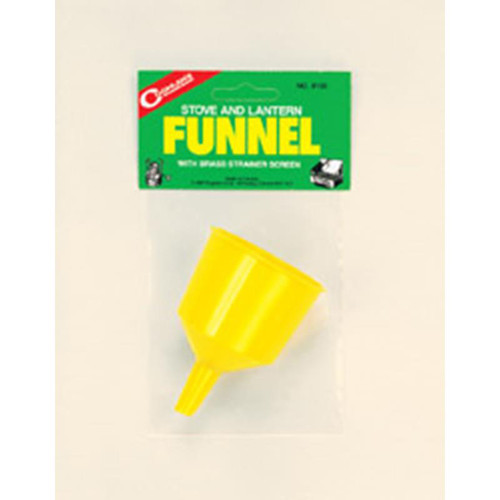This image depicts a full-color photograph of a packaged funnel, likely intended for camping use, specifically for refilling stoves and lanterns. The funnel, made of hard yellow plastic, is housed within a black cellophane wrapper and attached to a green cardboard tag. The upper section of the tag showcases the product name with "Stove and Lantern" in white text followed by "Funnel" in bright yellow uppercase letters. A red ribbon with white text adorns the upper left corner of the packaging, although the specific writing is unclear. The backdrop of the image is a cream-colored, possibly scanned surface. The photo appears somewhat poorly done but retains enough detail to identify the product as a practical tool for outdoor cooking or vehicle maintenance.